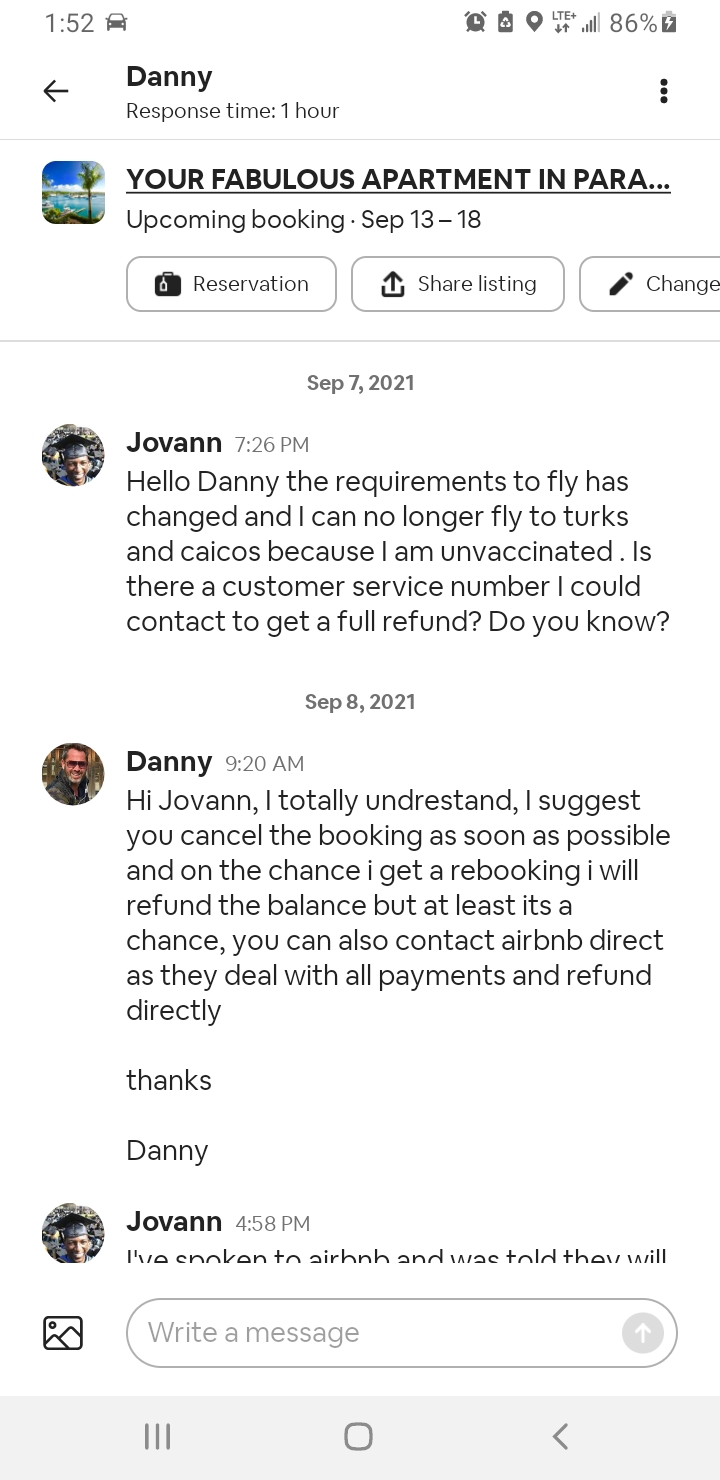**Descriptive Caption:**

In this screenshot, we see a conversation on a mobile app where Danny is discussing a booking for a luxurious apartment in Paris. The screen displays various options such as "Reservation," "Share," "Listen," and "Change." The booking is scheduled from September 13th to September 18th. 

The conversation itself started on September 7th, when Joe Vann messaged Danny at 7:26 AM, expressing a concern about changes in travel requirements preventing him from traveling to Turks and Caicos due to his vaccination status. He inquired about a customer service number to contact before leaving the hotel. 

The following day, Danny responded at 8:13 AM, advising Joe Vann to cancel the booking as soon as possible, with a note that there might be a chance for a refund depending on the rebooking policy of the service they are using, Airbnb. Danny also mentioned that contacting Airbnb directly might be helpful as they handle all payments and refunds.

A reply from Joe Vann at 4:58 PM is partially visible, indicating he spoke with Airbnb and received information about a potential refund, but the details are cut off in the image.

At the very top left of the screen, the device indicates car mode, with a time of 1:52 PM, active LTE connection, an alarm icon, and a battery being charged at 86%.

Both the conversation and the booking details reflect a complex situation involving travel changes and customer service interactions.